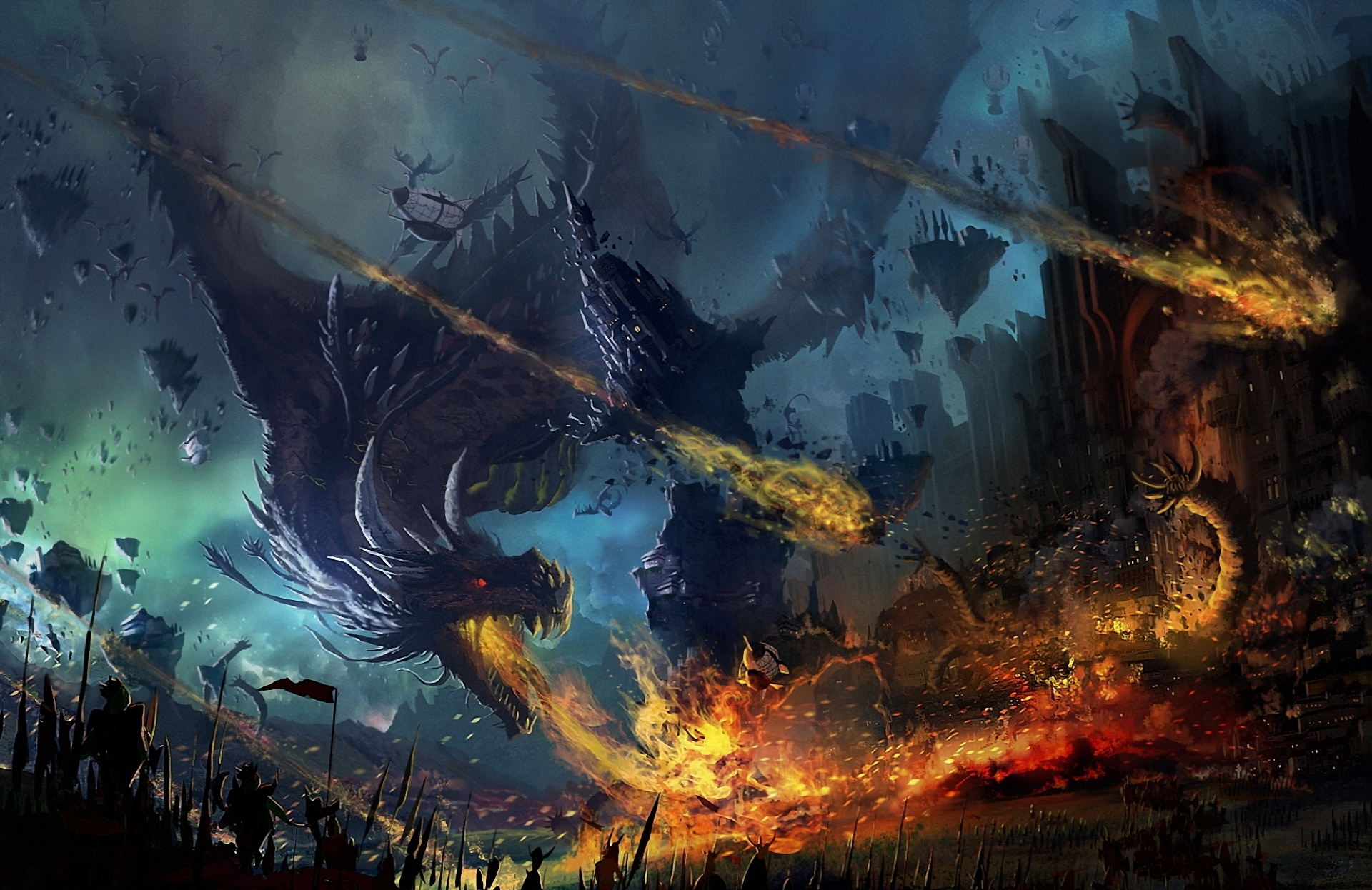In this striking animated image, a fierce dragon is depicted setting the ground ablaze. The dragon, with its imposing dark gray scales and one piercing red eye, dominates the center of the scene. Flames rage around it, casting an orange and red glow across the ground. To the left, a group of silhouetted figures brandish sharp weapons, their shapes backlit by the inferno. One of these figures waves a black flag with a greenish hue at its base. Beyond the dragon, the sky is a tumultuous blend of blue and gray, adding to the sense of chaos and destruction. On the right-hand side of the image, part of a brown castle is visible, partially obscured by the encroaching flames. The scene is a vivid portrayal of a mythical battle between human resilience and draconic fury.